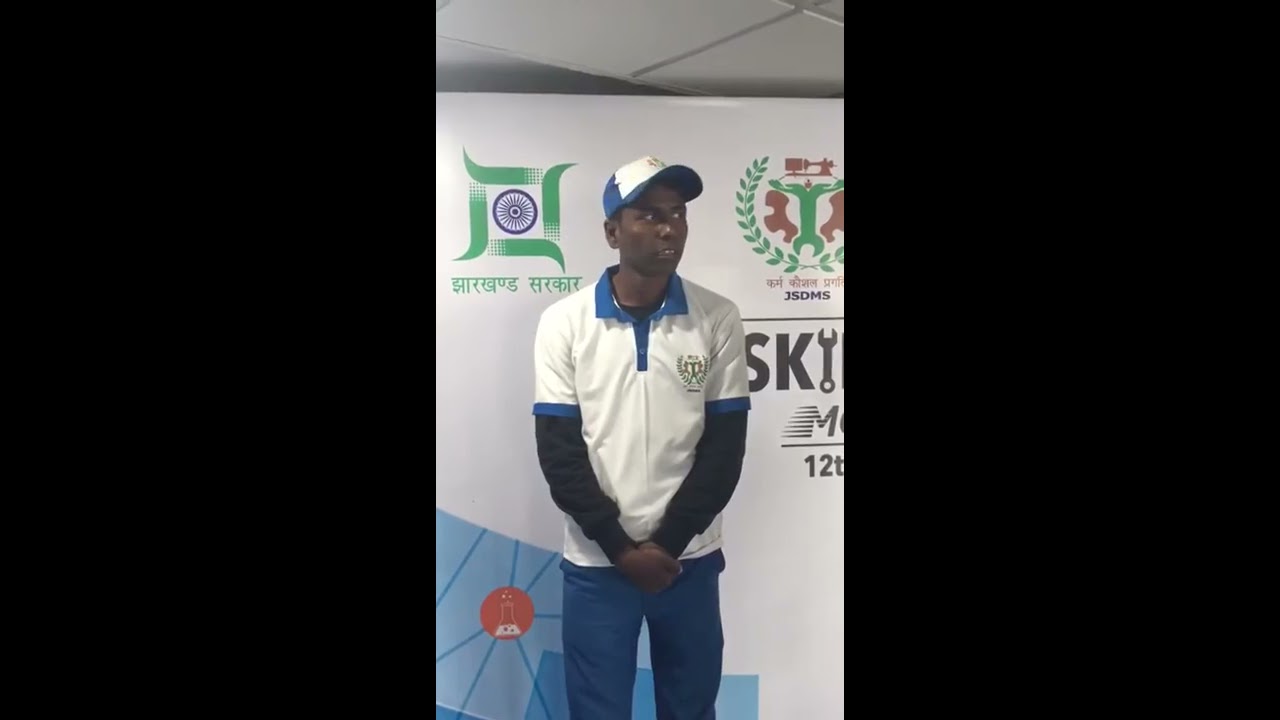The wide image is divided into three vertical sections, with the left and right thirds being completely black. In the center, a slim section features a dark-skinned African-American male. He is wearing a white short-sleeve polo shirt with blue collars and blue rims around the sleeves, over a black long-sleeve shirt. The man has on a white baseball cap with a blue brim and a blue back, and blue jeans that are visible to his knees. His pose shows him facing the camera, but looking off to his left, with his hands down by his crotch area.

The background behind him includes a drop ceiling with white tiles and a banner with multiple logos and symbols. One logo has a green wave pattern with a blue wheel in the middle. Another shows a wrench next to the letters "SK," and there are additional icons including one that looks like a man lifting with a gear and laurels, a logo with a swirly design, and a small red logo in the bottom right corner. The logo on his hat and shirt features a green wrench-like symbol with vine-like elements. The setting suggests a presentation or event possibly related to tools or mechanical subjects.